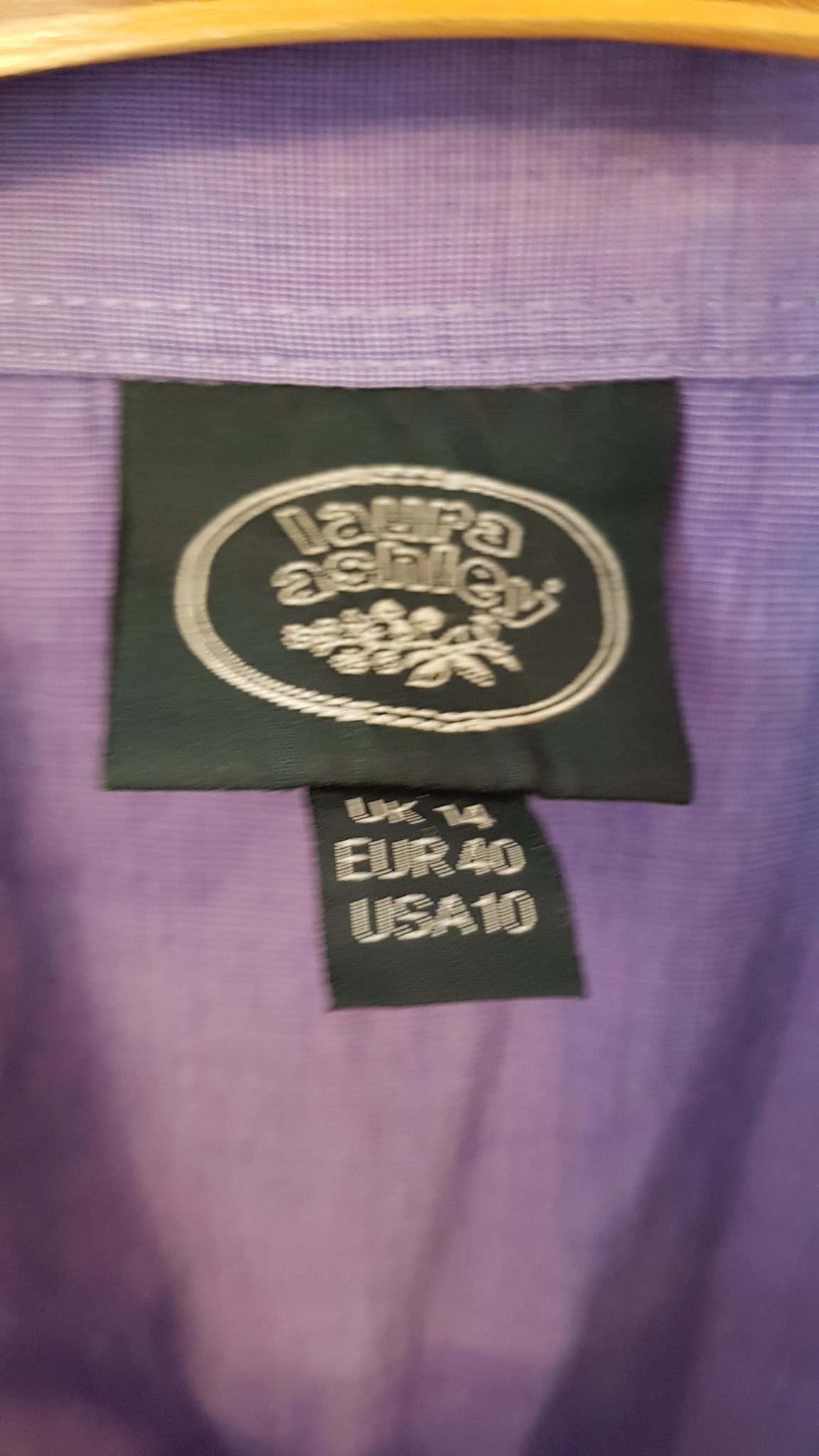The photograph captures a slightly blurry, detailed close-up of the inside collar area of a purple woven cotton shirt, branded Laura Ashley. The fabric appears a bit wrinkled and faded, with a faint pattern visible and white stitching along the collar seam. A light wooden curved hanger is positioned across the top of the image. Centrally located on the collar seam is a black tag featuring a gold oval with the Laura Ashley logo and decorative gold leaves. Below this main tag, a smaller black tag displays the clothing size information: UK 14, EUR 40, USA 10.